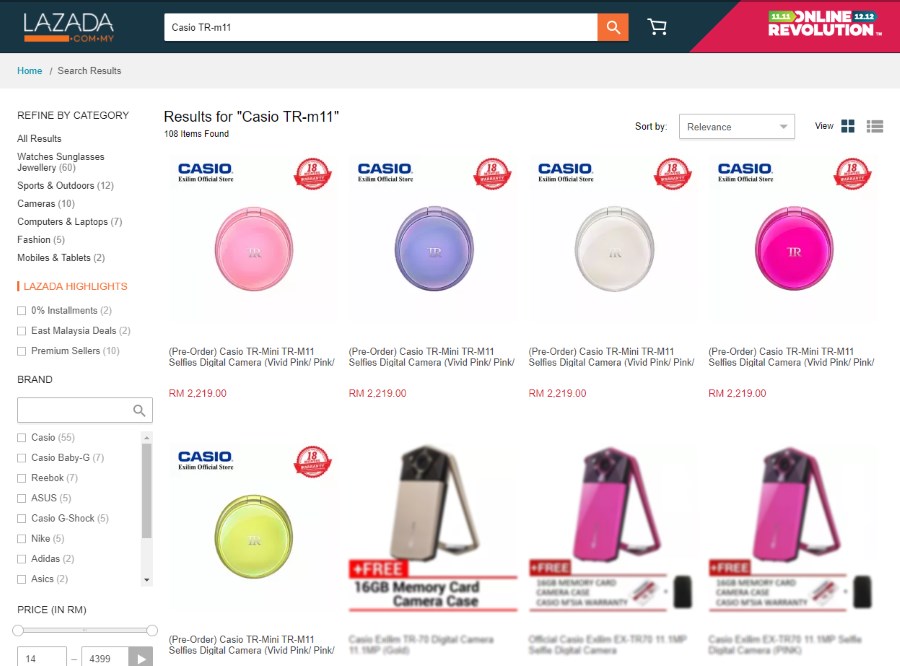This image is an advertisement from Lazada, a company specializing in the sale of electronic equipment. The focal point of the ad is a search bar where the term "Casiotr" has been entered, revealing a variety of results, particularly highlighting the M11 model. The search results showcase a spectrum of color options including pink, purple, white, lime green, and darker pink. The ad also mentions that these items are available for pre-order.

Additionally, the advertisement displays images of complementary items, such as memory cards and camera cases, which are offered for free. It includes a section for refining search results by category—spanning watches, sunglasses, cameras, and mobile devices and tablets. Users can also filter products by brand with featured names like Casio, Reebok, Asus, Nike, Adidas, and Asics.

Lazada seems to be promoting an "Online Revolution", suggesting that their platform may operate exclusively online. The ad also features a shopping cart icon, allowing users to add and save items, presumably with an unseen checkout process. The overall image effectively demonstrates the functionality of the search bar and the diverse array of available choices.